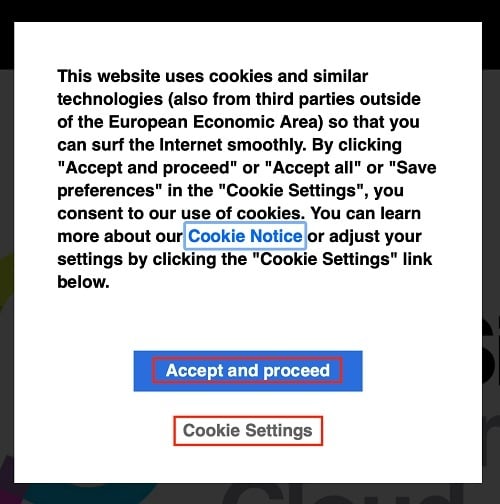The image depicts a notification about cookie usage within a stylized square format. The outermost square features a black background with a distinct border: thicker on the top and bottom edges and thinner on the left and right sides. Encased within this border is a central white square containing the main text of the message.

The message informs users about the website's use of cookies and similar technologies, mentioning explicitly that these may include third-party cookies outside the European Economic Area (abbreviated EEA).

The text explains that by interacting with the notification—specifically, by clicking "Accept and Proceed", "Accept All", or "Save Preferences" (all phrases are in quotations)—users consent to the use of cookies. There is an option to learn more about the cookie policy, highlighted by blue text enclosed within a blue rectangle, noted as "cookie notice."

At the bottom of the notification, a blue banner contains the call-to-action buttons: "Accept and Proceed" is in white text within a blue rectangle outlined in red, and "Cookie Settings" appears separately, also with a red border. This banner provides users with the option to adjust their cookie preferences directly.